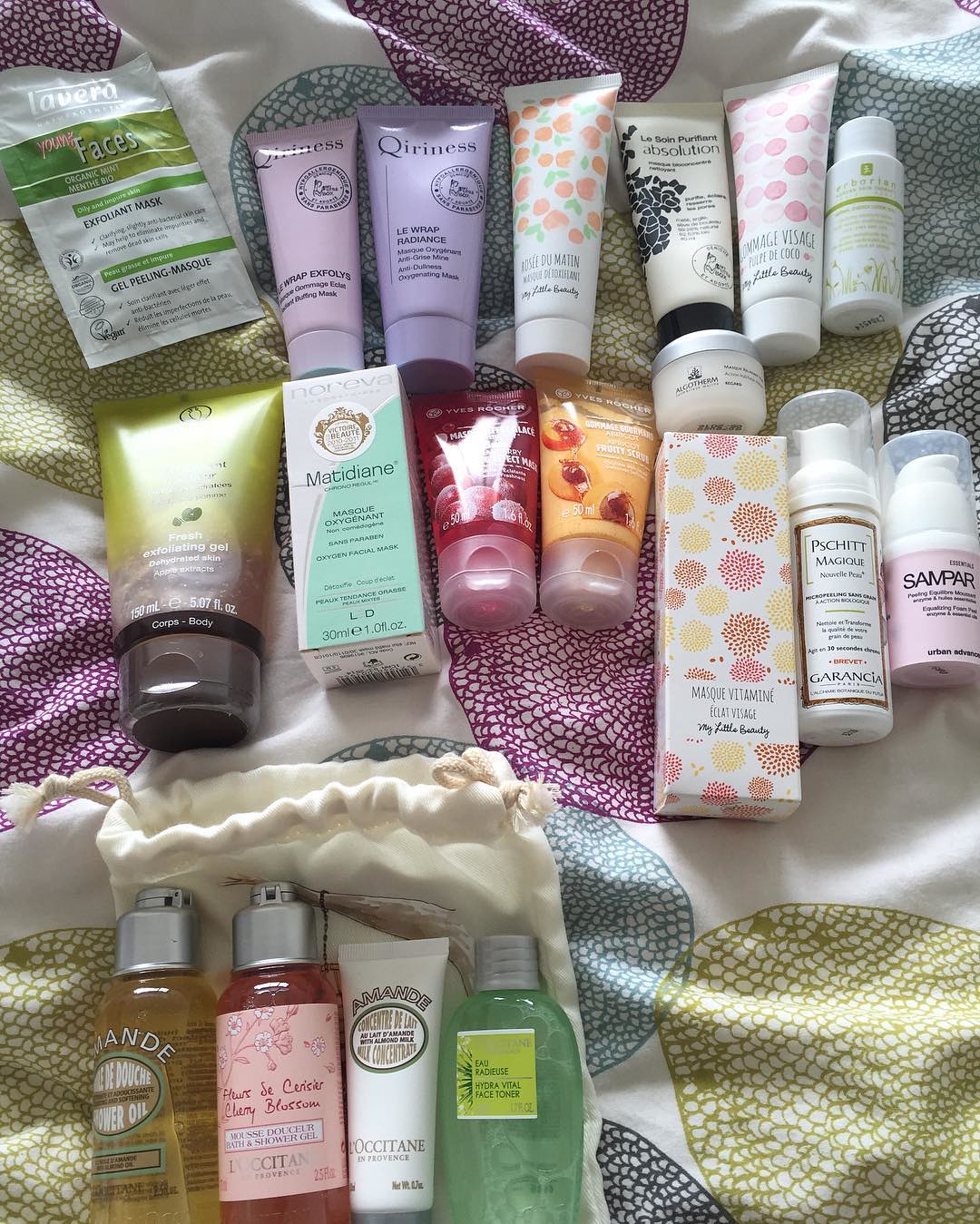A meticulously arranged collection of cosmetics and personal care products is displayed on a white cloth with a vibrant circle pattern printed in purple, green, yellow, and black. The products are organized in two rows, with additional items placed on a white muslin drawstring bag at the bottom.

Starting from the top left of the first row, there is a pouch labeled "Avira Youth Faces Exfoliant Mask and Gel Peeling Mask." Following this, moving right, are two similar-looking tubes in violet and purple, both branded with "Queerness" and adorned with unreadable medallions. The violet tube is labeled "Wrap Exfoliants," while the purple one reads "Le Wrap Radiance." Next is a white squeeze tube featuring an image of red fruit with green leaves, likely roses, and labeled "Rose du Matin, My Little Beauty."

Adjacent to this is another white tube with a black cap, decorated with black flower petals and the text "Absolution." Proceeding further right is yet another white tube, this time with pink and red dots, labeled "Fromage Visage, Something de Coco, My Little Beauty." A white bottle with a gold writing follows, though the text is illegible.

In the second row, there is a large wide squeeze tube labeled "Fresh Exfoliating Gel," 150 milliliters (5.07 fluid ounces), with English and French wording "corpse.body." Next is a small cardboard box bearing the brand name "Noriva" and the label "Matadion Mask Oxygenant." A clear squeeze bottle with red gel and pictures of red grapes is partially legible, displaying the words "mask" and possibly "Yves Robert," with a volume of 50 milliliters (1.6 fluid ounces).

Another clear tube, presumably with an overprint of half peaches on a cream background, similarly hints at the brand "Yves Roger" and the product name "fruit scrub." Following that is a white box adorned with yellow, red, and orange flowers made of little dots, labeled "Mask Vitamine visage, My Little Beauty." The row concludes with two white squeeze bottles labeled "Mask" and "Sampar."

Finally, atop the white muslin drawstring bag at the bottom are two bottles with flip caps resembling hand soap or shower gel, a white squeeze tube labeled "Amanda, something concentrate," and a clear bottle containing green liquid labeled "Hydrovital Face Toner."